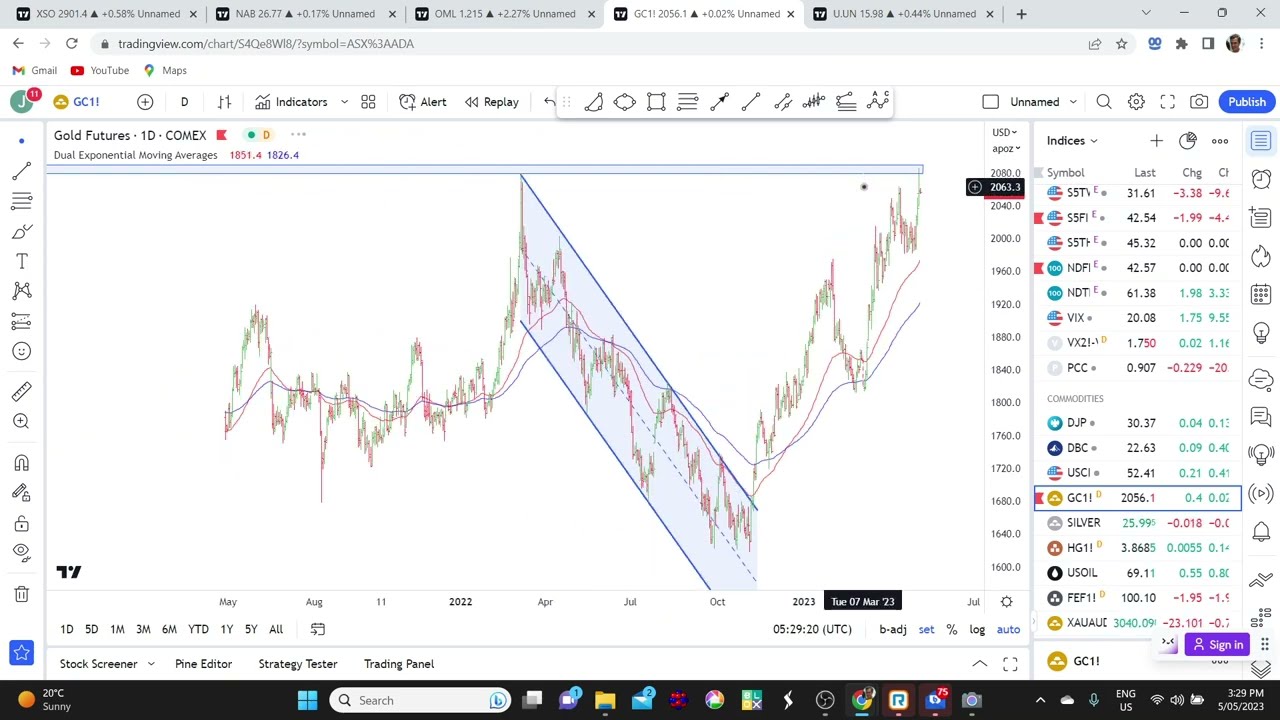The image displays a Windows desktop showcasing the TradingView website, evident from the five open browser tabs, all with the same logo, the fourth of which is highlighted. The main part of the screen is dominated by a detailed line graph, likely representing stock or gold futures fluctuations from 2021 to 2024, marked by green and red lines indicating performance changes. A blue diagonal highlight distinguishes the pre-2023 and post-2023 periods. To the right of the graph, an indexed list of stock tickers is visible, presenting various acronyms and numerical data to track market changes.